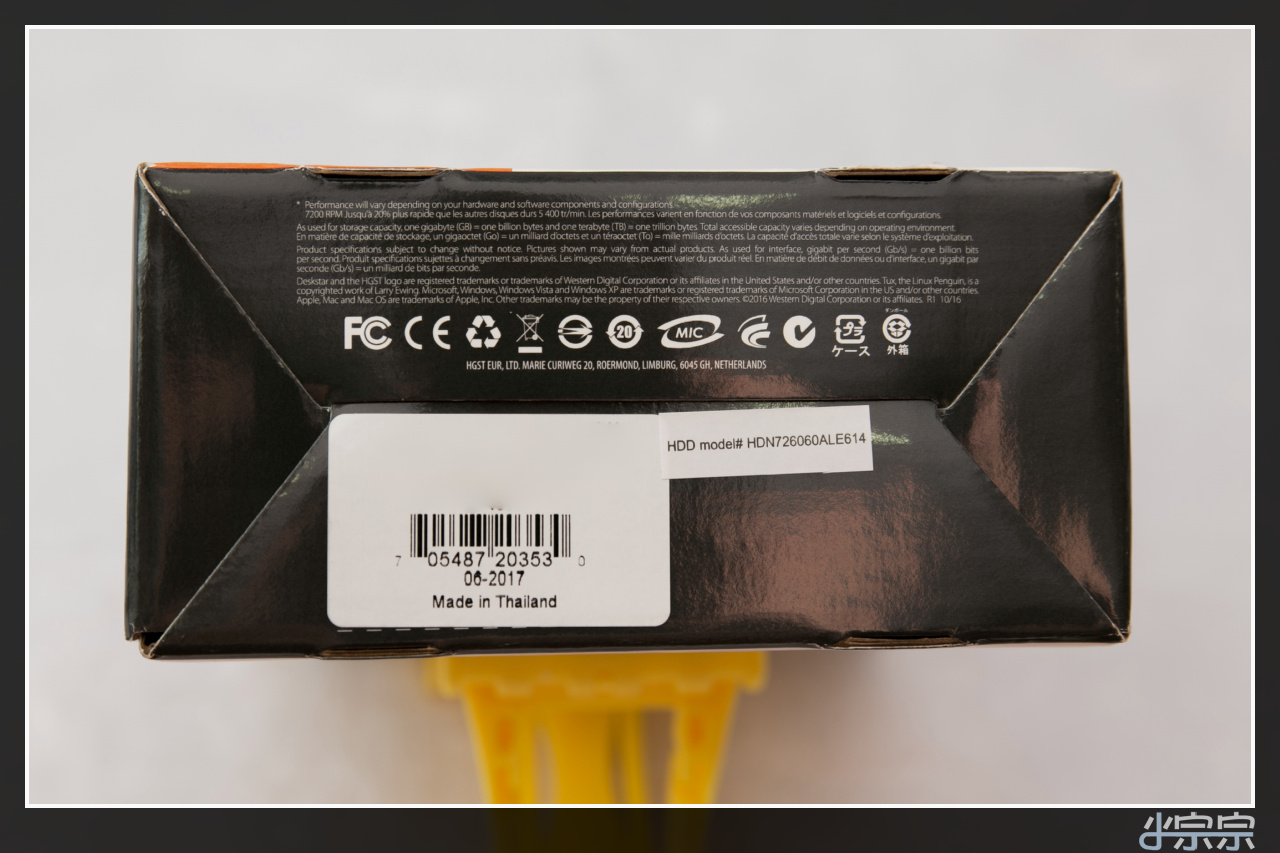This image depicts the bottom of a black box with intricate folding flaps that interlock without the use of tape. The text "Made in Thailand" is prominently printed alongside a scannable SKU barcode. The bottom is adorned with various white symbols and a detailed paragraph of white text. Additionally, there appears to be yellow substance either emerging from or dripping from the box, though its exact nature is unclear. A distinctive mark, possibly Asian writing or a unique symbol, is visible in the bottom right-hand corner.